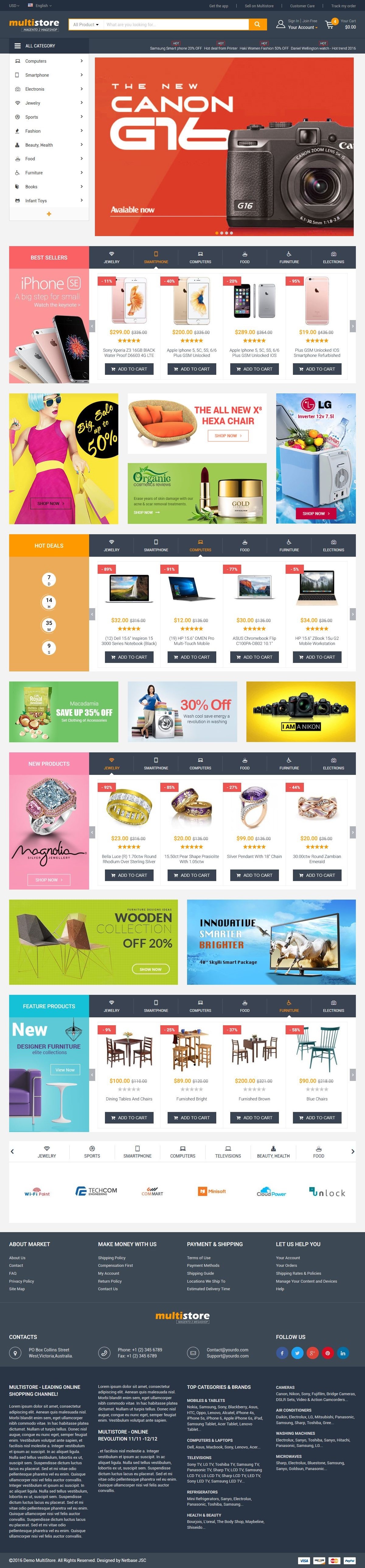An image of a web page appears small and blurry, making it difficult to discern specific details. The top of the page features a black and orange background with a search box prominently displayed. On the left side of the page is a menu, although the specific options are unclear. To the right, there is a red box containing an image of a camera labeled "Canon something." Above this, there are images of four different smartphones stacked on top of each other. Further down, there is a picture of a person wearing a purple shirt and a matching purple skirt, along with some household furniture including chairs, tables resembling a kitchen set, a sofa, and a coffee table set. At the bottom of the page is a block of text accompanied by social media icons for Facebook, Twitter, and Google Plus on the right side.